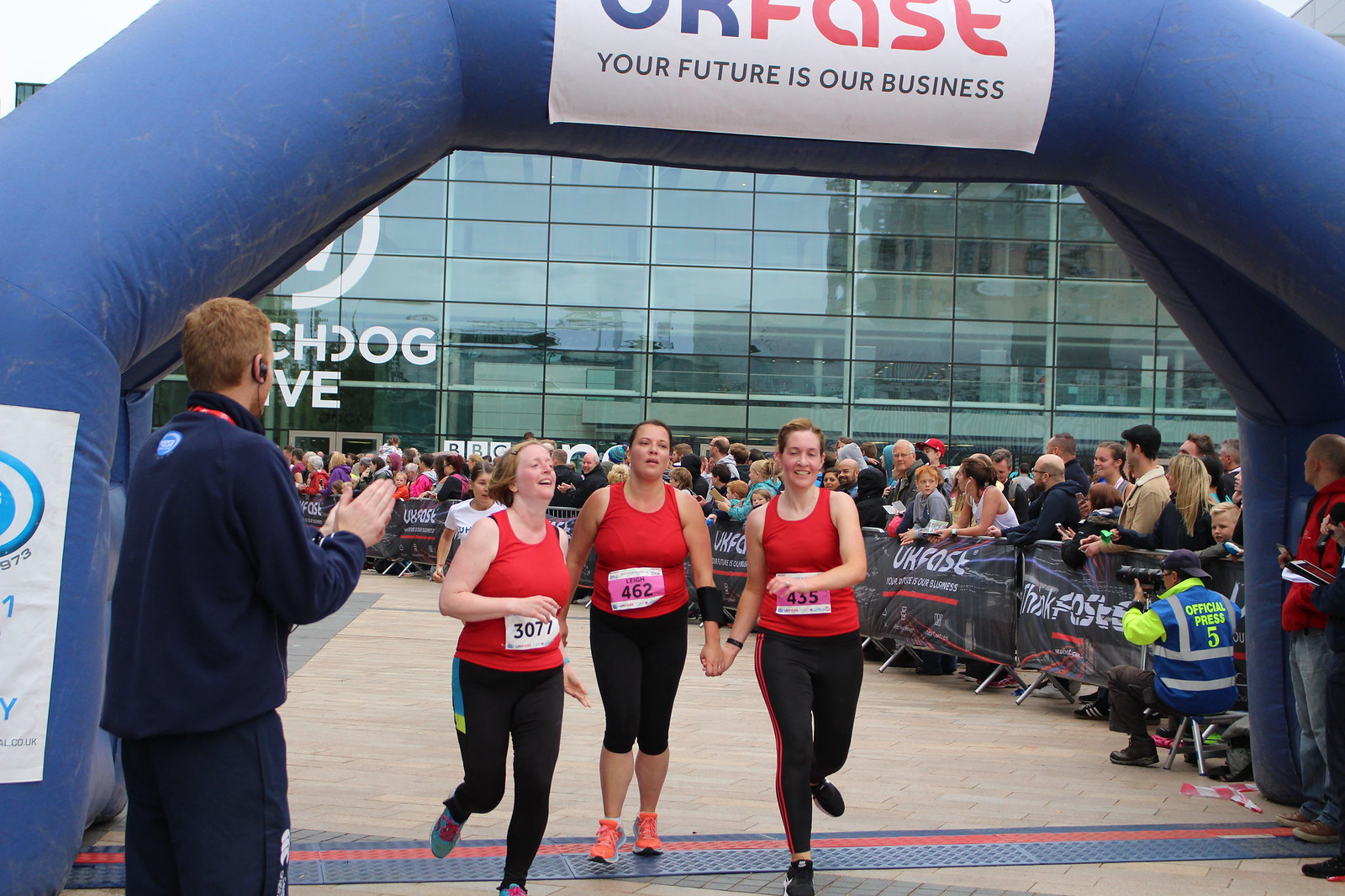In the vibrant scene of a daytime marathon, three female runners, all wearing red tank tops and black leggings, triumphantly cross an inflatable blue finish line arch together, holding hands. Above them, the arch features the slogan "Your Future is Our Business." Their bib numbers, 3077, 462, and 435, are visible as they smile despite their exhaustion. Surrounding them is a lively crowd of spectators, eagerly clapping and cheering behind barricaded fences against the backdrop of a gleaming glass-fronted building. Closely observing the finish, a man in a long-sleeved blue shirt, blue pants, and a red lanyard looks on attentively, equipped with an earpiece and a shock of red hair. Off to the left, an official press photographer captures the moment, marked by his blue vest and camera.